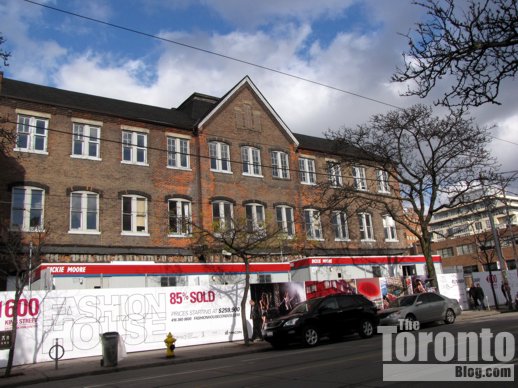The image depicts a lively city street scene. Dominating the view is a large, three-story brown brick building with a peaked roof in the center and numerous windows—11 on each of the second and third stories. The ground floor is obscured by a barricade in front, featuring a billboard that reads "Fashion House, 85% Sold". In front of this, there are two cream-colored trailers or buses with red tops and illegible writing on them. Along the street, two cars are parked, one black and one gray. The street is lined with a couple of bare trees, a fire hydrant, and a garbage can. Another building is visible down the street, and several people are scattered throughout the background. Overhead, an electrical line crisscrosses a blue sky with white clouds. The bottom right-hand corner of the image bears the text "thetorontoblog.com" in light gray lettering.